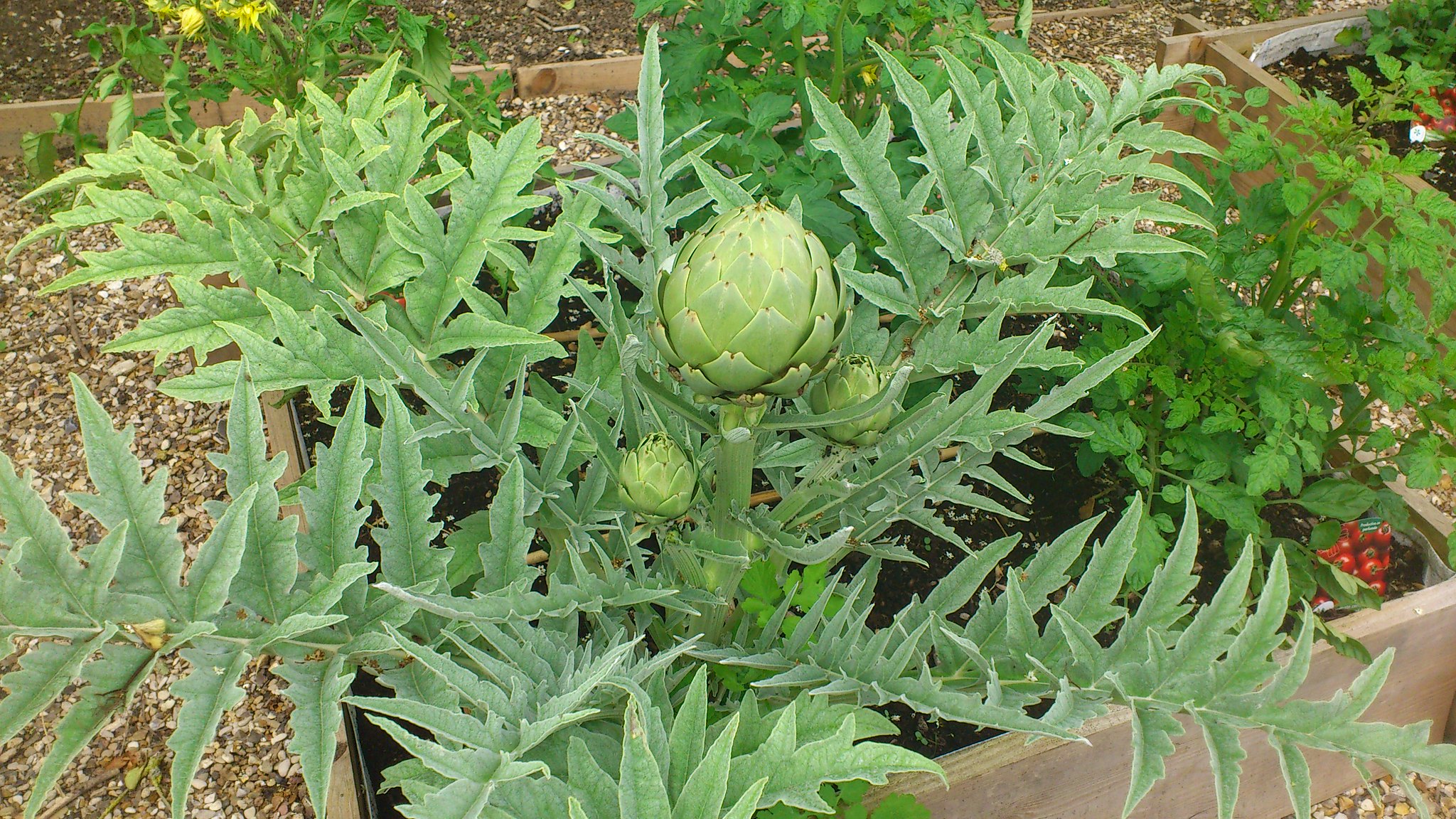This photograph captures a close-up of a large, green artichoke plant anchored in a square planter constructed from four light brown two-by-fours. The central feature of the plant is a thick stem supporting three artichokes—one large in the center and two smaller ones flanking it. The plant's numerous triangular leaves extend outward robustly from the base. The planter, a grayish-olive wooden box, houses rich, dark soil. Adjacent to the main artichoke plant on the right is a smaller plant with darker leaves. A little sign next to this secondary plant suggests it might be a tomato plant, depicted with small red tomatoes. The background of the scene includes a mixture of pebbles and dirt, interspersed with another similar wooden planter to the right. The entire area is enclosed, showcasing a natural palette of light brown, gray, and green colors.